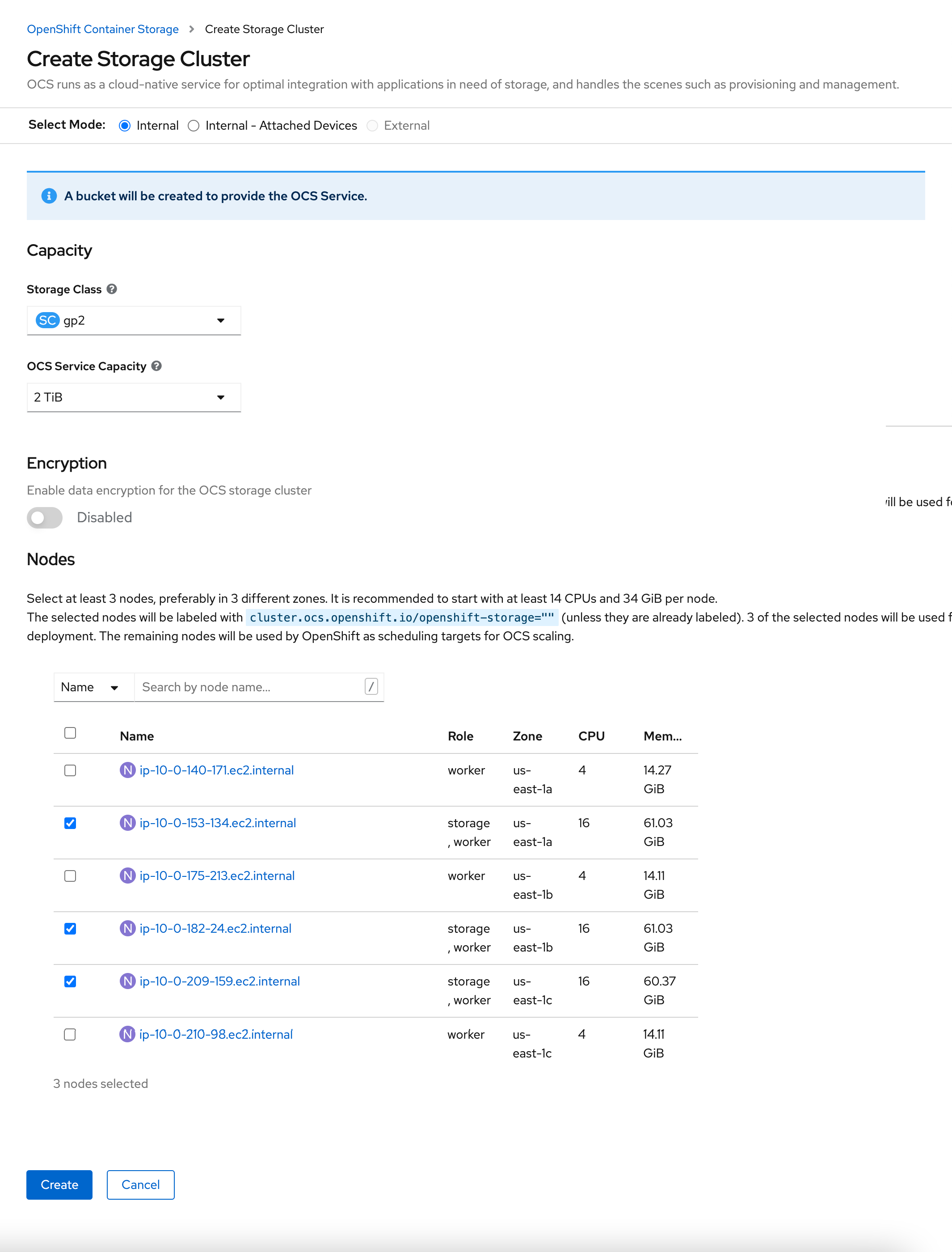The screenshot captures a webpage from some kind of application management program or website. At the top, the heading "Create Storage Cluster" is displayed in black, and right above it, the title "OpenShift Container Storage" is prominently highlighted in blue, followed by the subheading "Create Storage Cluster."

An explanatory paragraph follows, stating, "OCS runs as a cloud-native service for optimal integration with applications in need of storage and handles the scenes with provisioning and management." Below this description, there is an option to select from different storage issues. The first option, labeled "Internal," is selected and marked with a blue circle. Two additional options are listed: "Internal - Attached Drives or Devices" and "External."

Directly beneath these options lies a horizontal blue bar accompanied by a thin blue line at the top. Adjacent to this bar is a small blue icon featuring an "i" inside it, indicating more information. The text informs the user that "A bucket will be created to provide the OCS services." The section continues with details about capacity, storage class, and OCS serving capacity.

Additionally, there's an encryption toggle switch that is currently disabled. Moving further down, the interface guides the user to select at least three nodes, ideally situated in three different zones. A list of names resembling IP addresses is displayed, with some of them checked off, indicating selection, while others remain unchecked.